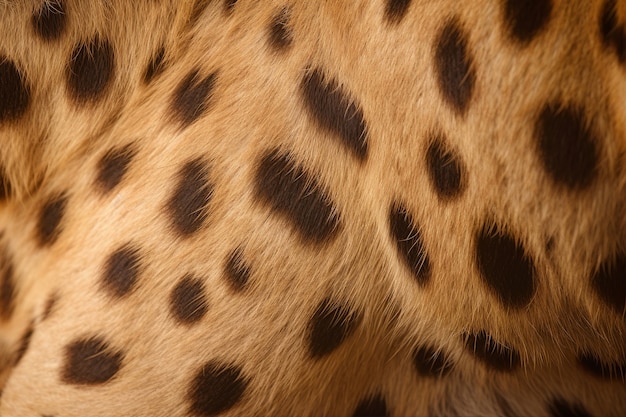This highly detailed close-up photograph showcases what appears to be a leopard's fur, though it could also be a realistic leopard-print fabric. The fur, or fabric, features a light brown or sandy-colored background, accentuated with an array of dark brown, coffee bean-colored spots that vary in size from small dots to larger patches. The fibers of the fur seem almost wispy and slightly long, giving the illusion of the soft texture of an actual leopard’s coat. The camera captures this texture and pattern up-close, filling the entire frame with no other elements visible. Slight creases in the fur suggest the presence of a limb, hinting at the possibility that this could be part of an actual animal. The detailed view emphasizes the rich, intricate pattern extending from the top left to the bottom right of the image.